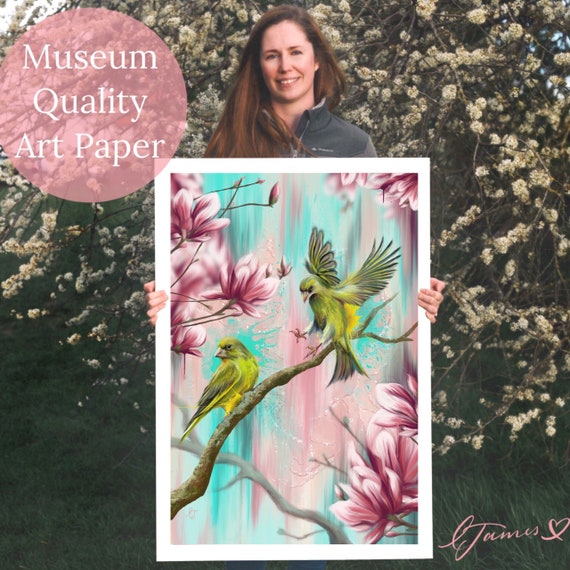The image is an advertisement for art paper, prominently featuring a logo in the upper left corner, a pink circle with white text that reads "Museum Quality Art Paper." In the lower right corner, there is a name, possibly "ETAMES," accompanied by a heart symbol. The background consists of bushes and trees adorned with light yellow flowers that resemble lilacs.

Central to the image is a white woman, with long brown hair flowing down her right shoulder, dressed in a gray jacket. She is standing in a grassy field with a large plant featuring white flowers behind her. She holds a large portrait, approximately three feet high and two feet wide, with both hands. The portrait features two green birds; one bird has its wings outstretched while the other is perched on a branch. The scene is decorated with pink flowers and set against a background of pink and blue flowing colors. The woman has a partial smile and her head is tilted slightly to the right.